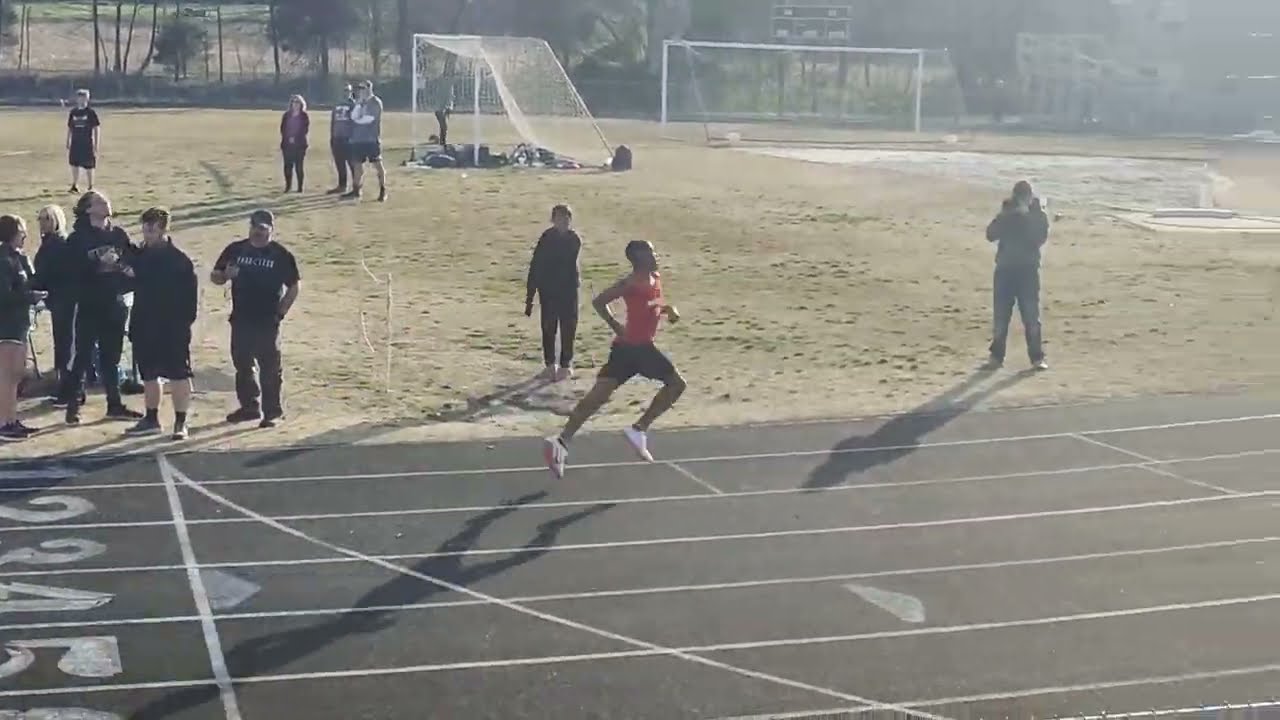The photograph captures a dynamic scene of a runner in mid-stride on an outdoor track, foregrounded by extensive detail. The runner, clad in a red sleeveless top, black shorts, and white sneakers, appears to be momentarily airborne as he advances down the brown track marked with white lanes. The track encircles a field patch that has green but sparse vegetation, hinting at an autumn day. On the trackside, multiple spectators can be seen dispersed: a group of five or six individuals on the left and two more to the right, with additional people in the distance. Notably, there is a man in a black hoodie with a white stripe who gazes upwards. The background is framed by trees and two white soccer nets, indicating that the area might also serve as a multi-purpose sports field. Also noticeable is a young boy in a black t-shirt and shorts. This vibrant snapshot is teeming with life as onlookers either watch the runner or engage in their own activities, adding depth and context to the image.